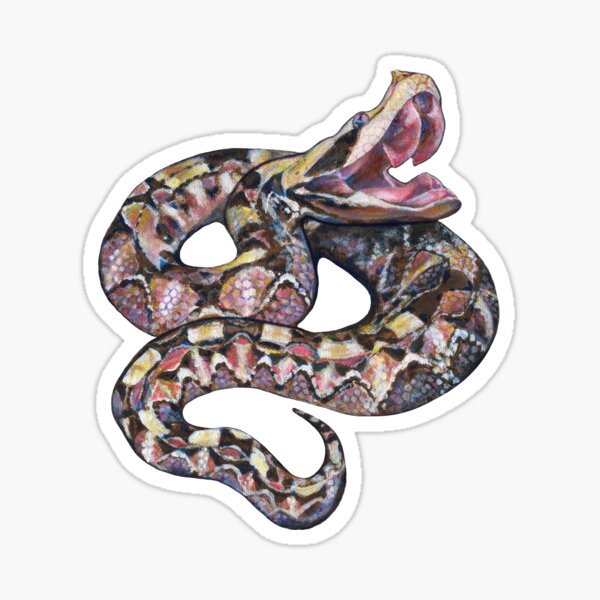This image features a vibrant, detailed drawing of a snake that's coiled in an S-shape. The upper portion of the snake showcases its mouth wide open, revealing visible fangs curving down from the roof of its mouth. Its head, positioned in the upper right corner, features a striking blue eye and a mix of green and black coloration. The snake's scales display a stunning array of patterns and colors—whites, pinks, yellows, and hints of gray—with intricate designs including spots, squares, and triangles. The tail is notably curved upward, devoid of a rattler, adding to its distinct appearance. The entire snake is outlined in white against a very light gray background, highlighting its artistic, almost cartoonish nature. The detailed texture of the snake's belly resembles pebbled diamonds, and it exudes a scaly look throughout. This artwork conveys both a sense of vibrancy and intricate craftsmanship, capturing the viewer's attention through its elaborate and colorful design.